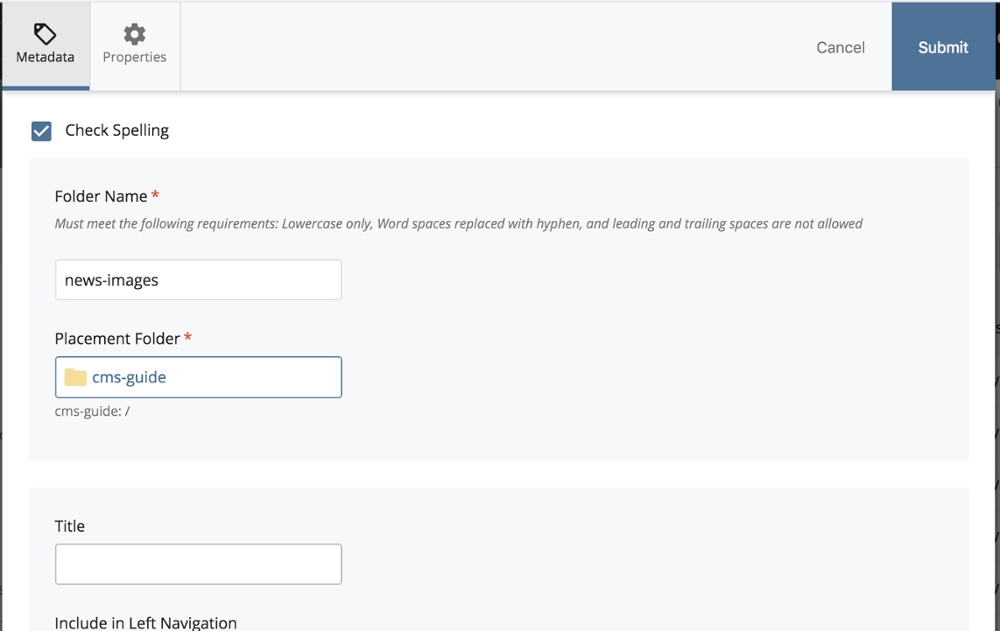In the screenshot, the title bar displays several elements: a "Metadata" button, a "Properties" button accompanied by a setup icon, and on the far right, a "Cancel" button followed by a "Submit" button enclosed within a blue rectangular box. Directly below the title bar is a "Check Menu" item labeled "Check Spelling." 

Further down, there is a light gray rectangle containing a label "Folder Name" marked with a red asterisk, indicating that this field is required. Beneath this label, there are instructions to fill in the folder name. Following this, there is a white input box pre-filled with the text "news-images."

Next, there is another label, "Placement Folder," featuring capitalized initials (P and F) and a red asterisk. Alongside it is an input box with a white manila folder icon and the text "CMS-guide." Below this input field, the path "CMS-guide:\" is displayed.

Further down, the image includes another light gray rectangular box with the label "Title," accompanied by a required field asterisk. Beneath this label is an empty white rectangle for user input.

This descriptive walkthrough captures the detailed layout and contents of the image, highlighting the various buttons, input fields, labels, and instructions present on the interface.